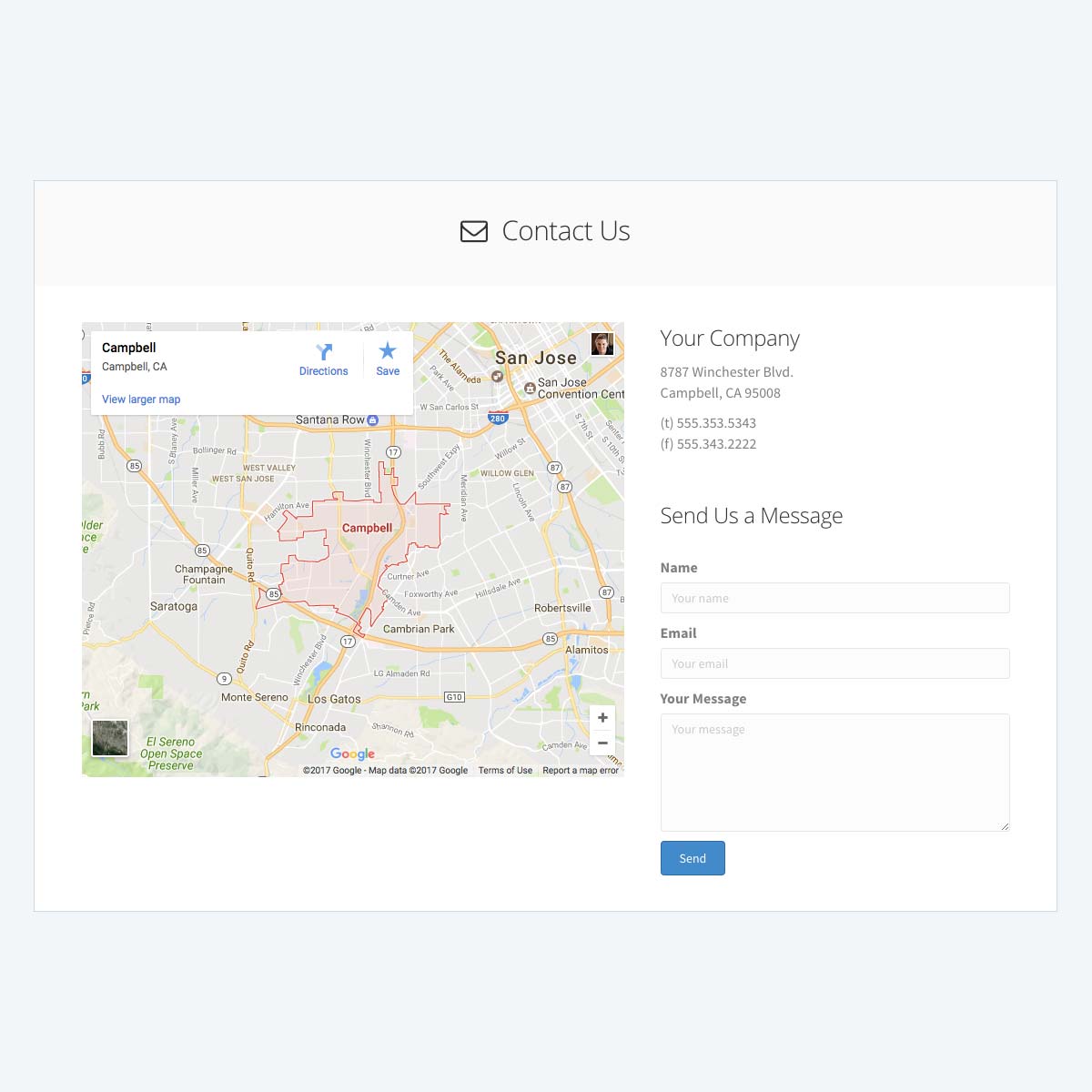This appears to be a screenshot of a "Contact Us" page from a website. The main layout consists of a pale bluish-gray background with a central white box outlined with a tan strip at the top. The top of the white box features a black "Contact Us" heading accompanied by an envelope icon.

Below this heading, there is an embedded Google Maps image dated 2017, indicating terms of use and copyright information. The map predominantly features gray, gold, blue, and green colors, illustrating the streets of Campbell, California, which is confirmed by labels showing nearby San Jose. The map also highlights businesses, location pins, highway numbers, and a red-marked area indicating Campbell, CA.

Above the map, there is a white box labeled "Campbell, CA," offering options in blue text to "View Larger Map," "Directions," "Save," etc. Adjacent to the map, the address "Your Company, 8787 Winchester Boulevard, Campbell, California, 95038" is displayed, along with phone numbers "555-353-5343" and "555-343-2222."

Below the address details, there is a form titled "Send Us a Message," featuring text fields for "Name," "Email," and "Your Message," capped off with a blue-and-white "Send" button.